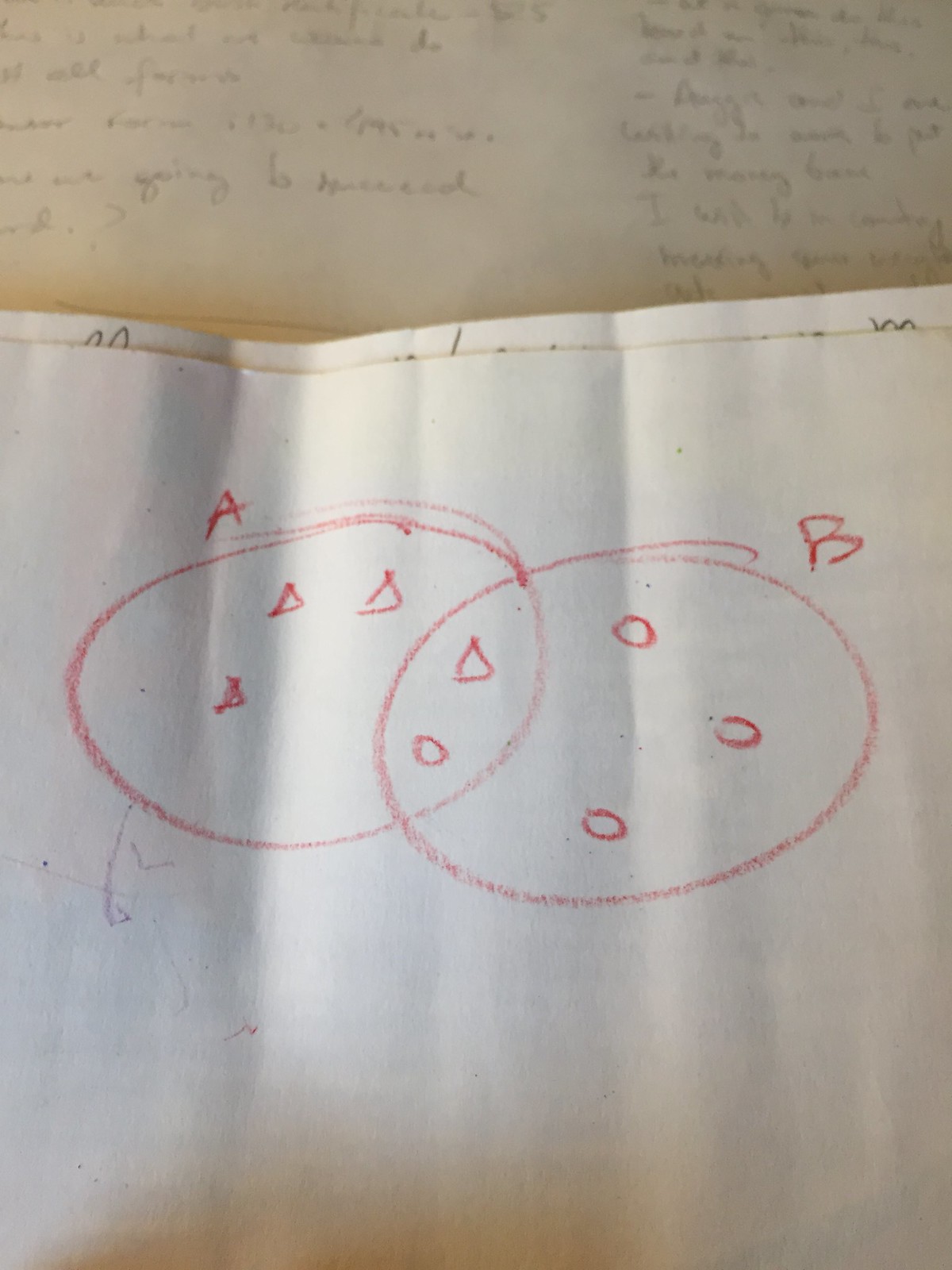The image features a diagram drawn on a sheet of white printer paper, resting atop another piece of paper. The secondary paper beneath exhibits faint pencil marks. Behind both sheets, a third paper is partially visible, containing handwriting in cursive, though the text is too distant to discern clearly.

On the primary sheet, the diagram consists of two interlocking circles. The left circle is labeled "A" and houses three triangles. The right circle, labeled "B" in Korean, contains three imperfect circles, each with a slight, irregular line protruding from their tops. At the intersection of circles A and B, there is one triangle and one circle, the latter sharing the same imperfect quality as those within circle B.

At the bottom of circle A, there's a peculiar gray, squiggly line. Additionally, a shadow extends upward from the bottom center of the image, suggesting the photograph was taken from a slightly elevated angle.